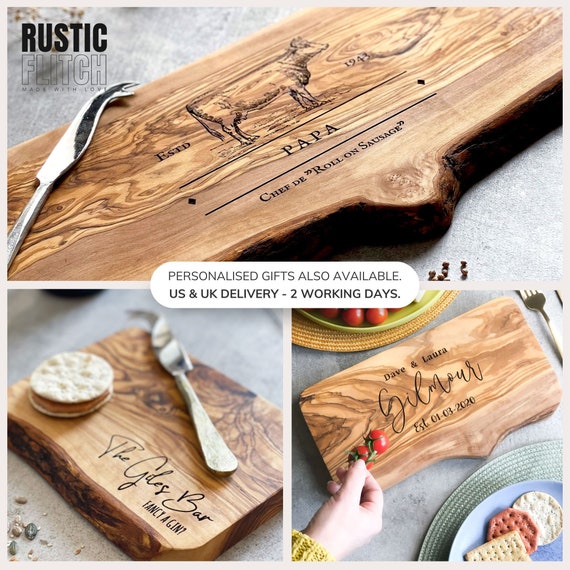This advertisement showcases personalized wood-burned cutting boards with a rustic aesthetic, available for delivery in the U.S. and U.K. within two working days. The photo is divided into three panes: the top pane occupies the entire upper half of the image, while the bottom half is split into two equal sections.

In the top section, the wooden cutting board prominently displays the brand name "Rustic Flitch." The board, crafted from dark, oak-like wood, features an engraved cow with the text "Papa Chef de Roll-on Sausage," accompanied by the year "ESTD 1943." A silver pronged butter knife rests atop this board.

The bottom left pane presents a smaller, equally rustic cutting board, showing the natural bark edge. This board holds three Ritz crackers spread with what seems to be peanut butter and another butter knife. Scripted beneath the crackers, faint cursive reads "the [something] bar."

In the bottom right pane, a marginally larger cutting board bears the inscription "David and Laura Gilmore," with an establishment date of "01-03-2020." A human hand extends from the lower left, holding cherry tomatoes over a green bowl, and in the lower right, a chic blue plate lies on a charger plate, holding three fancy crackers. 

Overall, the advertisement highlights the detailed and rustic charm of personalized wood-burned cutting boards suitable for unique gifts.